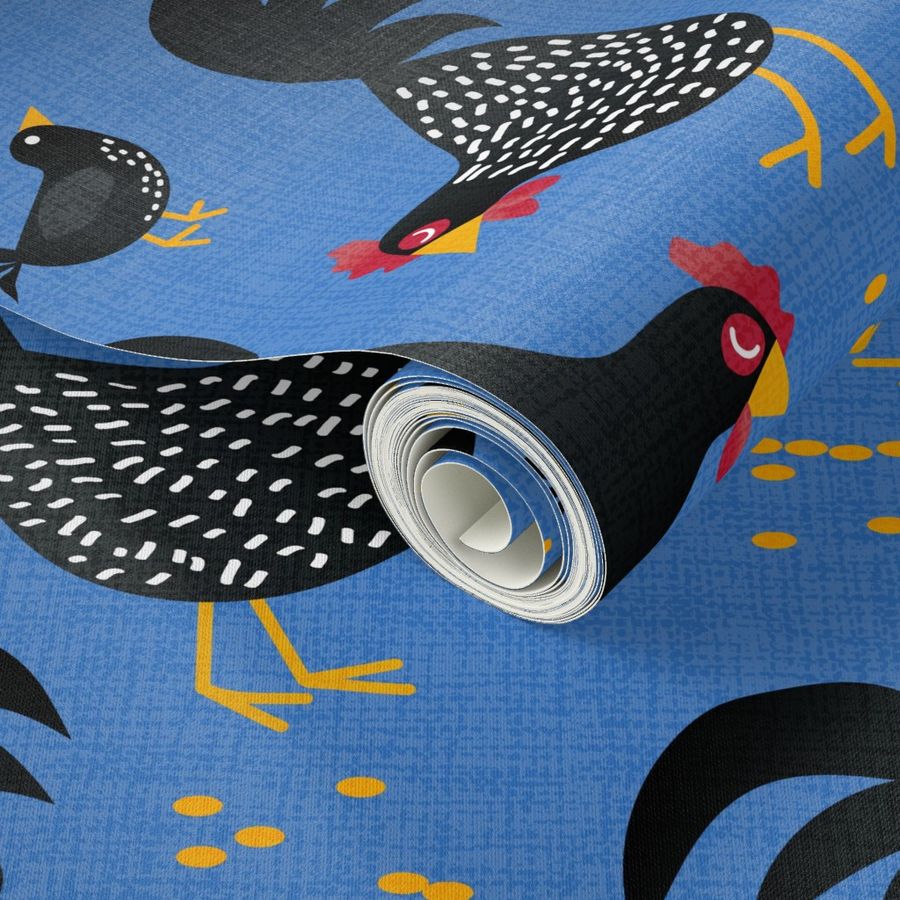This nearly square color photo features a rolled piece of vibrant, chicken-themed wallpaper set against a blue background and laid atop a flat sheet of the same design. The detailed wallpaper showcases black roosters adorned with white polka dots, yellow beaks, red combs, red beards, and bright yellow feet. These roosters have red eyes accented with U-shaped white slits for an artistic touch. Interspersed among the roosters are smaller black birds with yellow beaks, white dot eyes, yellow feet, and polka-dotted breasts. The arrangement of the birds is varied, with some depicted upside down and others shown from a head-up perspective. The colorful design is further enlivened by scattered yellow polka dots, contributing to its eye-catching, bright, and dynamic appearance.